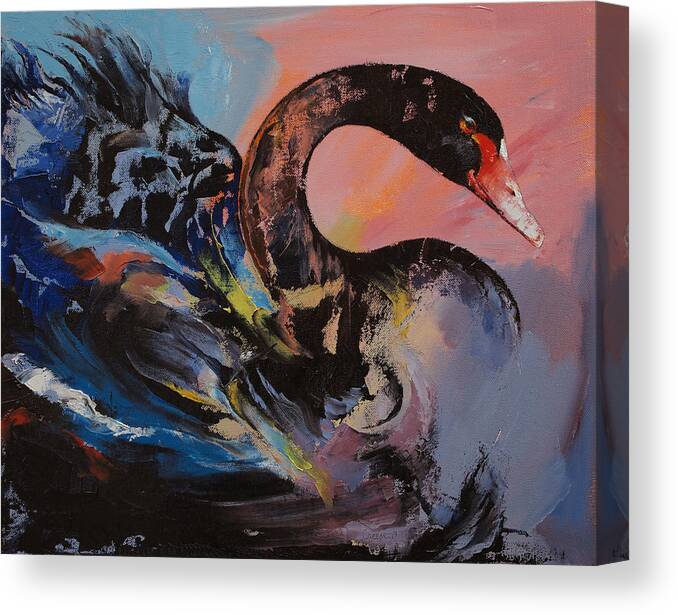This photograph showcases a canvas with a completed, highly stylized, impressionistic painting of a black swan. The swan, with its see-through head and detailed beak, gradually morphs into dynamic, swirling paint strokes forming its body and wings. These feathers mix black with an array of other colors, creating a vibrant yet ethereal effect. The painting is done with acrylic paints and is mounted on a solid white wall, casting a shadow to the side. The background is a vivid tapestry of various colors: the top left corner is dominated by reds and oranges, transitioning into pale blues and then darker, more saturated blues towards the bottom right. The hues also include deep purple, coral pink, and splashes of yellow, mimicking the chaotic yet beautiful essence of ocean waves, which subtly fade into and through the swan's feathers. The sharp edge of the canvas is visible on the right side of the photograph, hinting at the breadth of artistic expression contained within its borders.